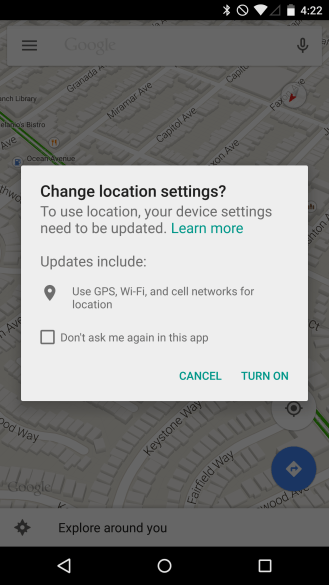This image displays a grayed-out map featuring various streets, including Miramar Avenue, Capitol Avenue, Granada Avenue, Keystone Way, and Fairfield Way. The map is not photorealistic; instead, it uses simple geometric shapes to indicate buildings, which are depicted as squares. Overlaying the map is a pop-up with a solid white background. The pop-up, written in black text, instructs the user to "Change location settings." It further explains, "To use location, your device settings need to be updated. Learn more," with "Learn more" highlighted in green text. The message continues, "Updates include use GPS, Wi-Fi, and cell phone networks for location." Beneath this text is a checkbox option, "Don't ask me again in this app." At the bottom right corner of the pop-up, there is a "Cancel" button and a "Turn On" button, the latter displayed in green text. Additionally, at the bottom of the map is a search bar labeled "Explore around you," indicating functionality for browsing local points of interest.